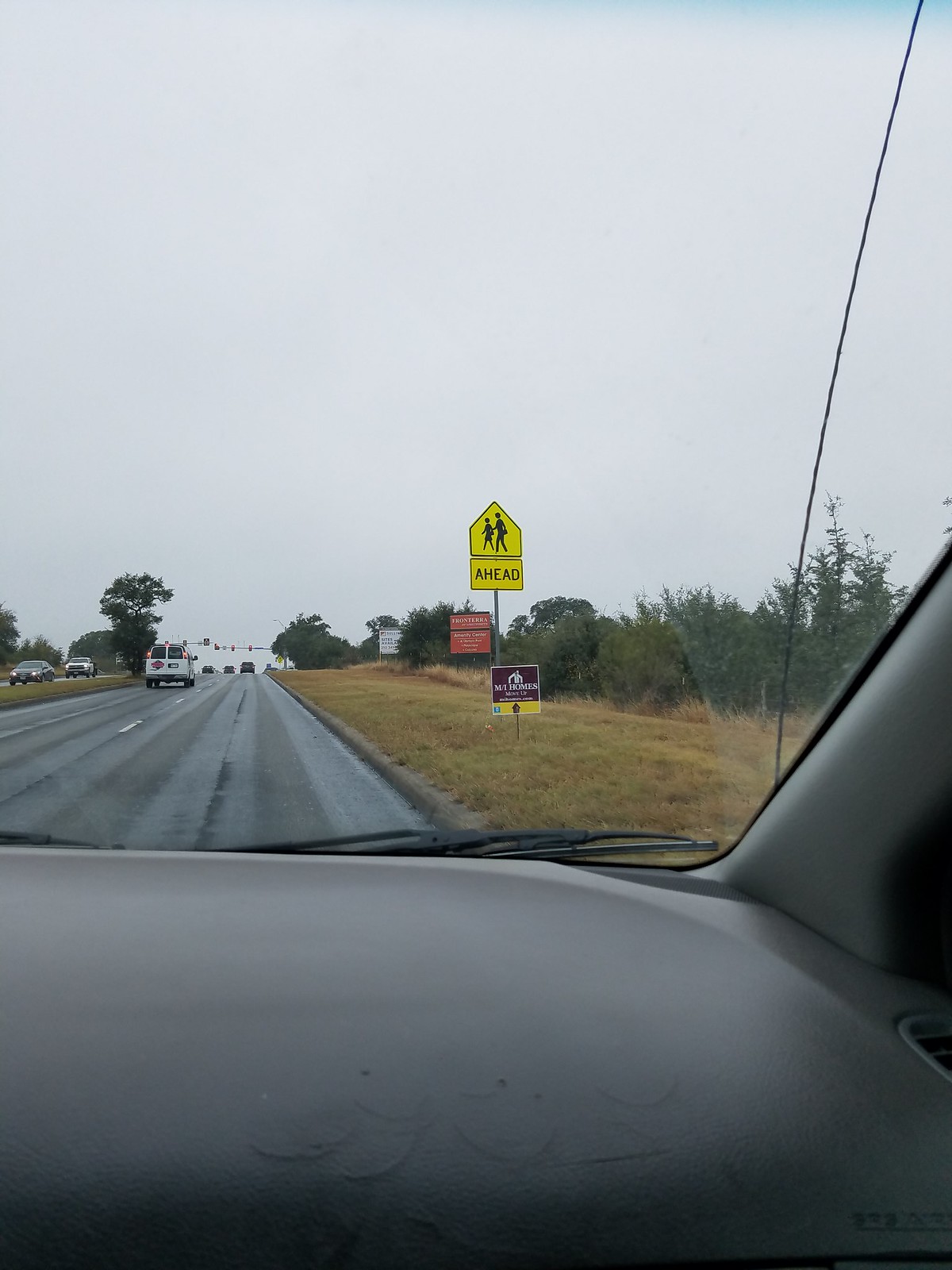The image depicts a street as seen through the dashboard of a vehicle. The flat, grayish dashboard frames the scene, with a glimpse of the windshield wipers visible on the lower edge. Along the periphery, part of the car's side is also in view. The road ahead appears to have three lanes, separated by a grassy median, with traffic coming from the opposite direction.

In the lane ahead, a white truck is visible. On the right side of the image, there's a grassy bank with a beige hue and a mix of various shrubs lining the edge. Several signs are positioned along the roadside: a yellow pedestrian crossing sign, a brown and yellow realtor sign, two red signs stacked together, and a white sign further in the distance. Additionally, traffic lights are seen far up ahead, indicating a controlled intersection.